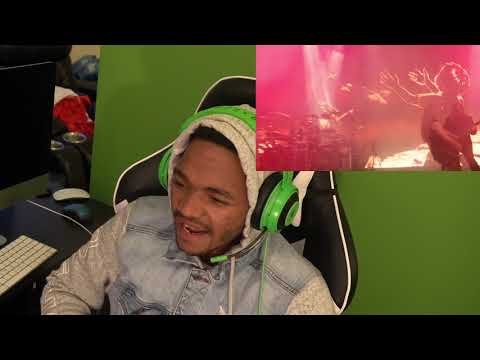In the image, an African American man sits at a black gaming desk, immersed in streaming, with an air of quiet focus. Dressed in a blue jean jacket layered over a grey hoodie, he also wears fluorescent green headphones equipped with an extendable mic. His seat is a black gaming chair accented by white stripes, and he is slightly smiling as he engages with his content. The green backdrop behind him serves as a green screen, enhancing his streaming setup. On the desk, in front of him, a computer monitor, white Apple keyboard, and black mouse are visible. In the upper right corner of the image, a FaceTime or reaction screen displays a vivid scene from a concert, with a crowd's hands raised in excitement and musicians performing, possibly indicating he is reacting live to a music video. The overall scene suggests a seasoned gamer or streamer engrossed in his online activities.